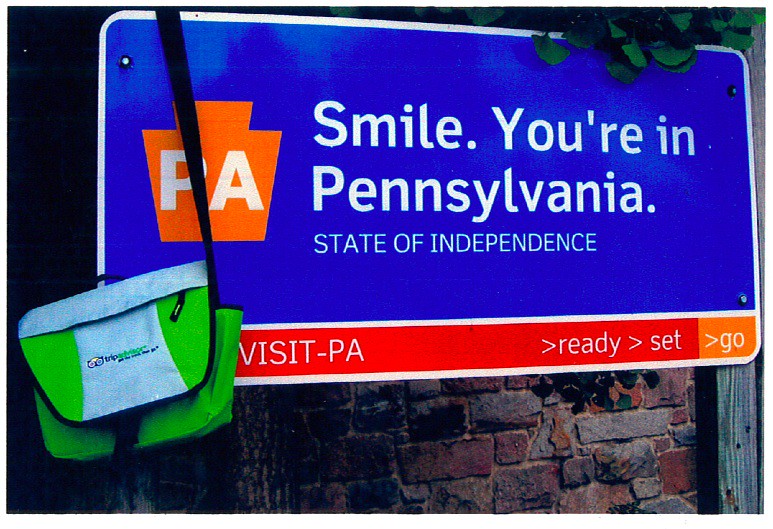In the image, there's a medium blue sign mounted on an old gray and red brick wall, possibly near a restaurant. The sign is outlined in white and prominently features the message "SMILE, YOU'RE IN PENNSYLVANIA, STATE OF INDEPENDENCE" in white lettering. At the top, there's an orange shield with "PA" in white letters, signifying Pennsylvania. Below this, an orange and red section contains the phrase "VISIT-PA" along with an arrow pointing right, followed by "READY" with another arrow, "SET" and finally "GO," in white letters on red and orange backgrounds. 

Hanging over the left side of the sign is a green and white insulated satchel with a black shoulder strap, bearing the TripAdvisor logo, which includes a green owl with unusual eyes. The bag appears to be looped over the sign, perhaps left there intentionally by someone for the original owner to reclaim. The sign is supported by two brown wooden posts, and surrounding the scene are green leaves, adding to the rustic outdoor setting.